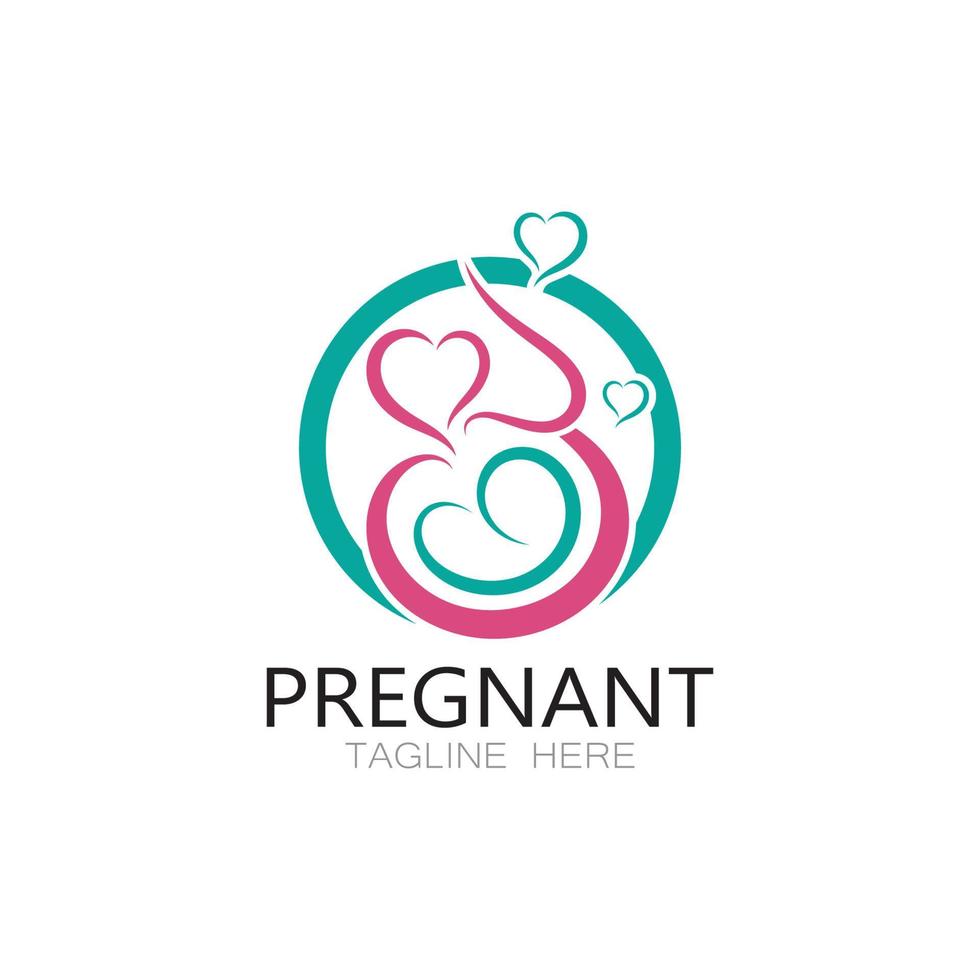The image is a white-background advertisement related to pregnancy, featuring a teal circle at its core. Radiating from the circle are various heart illustrations in both teal and pink. At the center, a dark pink line intersects with a teal heart shape, creating a layered effect. There's also a distinctive pink half-circle surrounding the teal heart in the middle. At the top right, a teal heart is pierced by a pink line extending from the circle. Below this central imagery, the word "PREGNANT" is prominently displayed in bold black text, followed by a placeholder tagline in smaller gray text. The overall design is elegant, with swirls and shapes that suggest the form of a pregnant woman cradling her belly, elegantly intertwining the hearts to evoke warmth and care, capturing the essence of pregnancy.